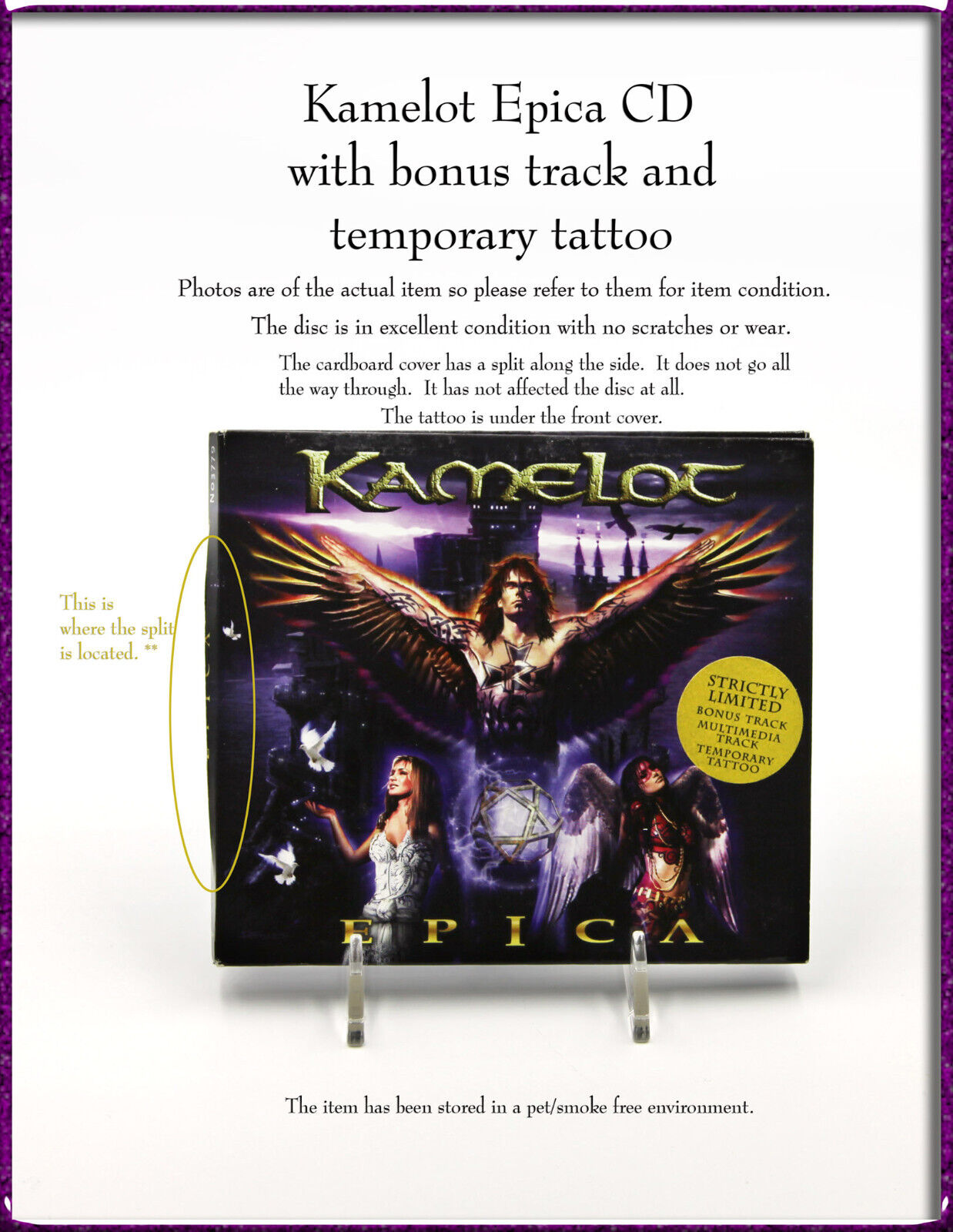This image is an advertisement for the Camelot "Epica" CD, featuring detailed descriptions and condition reports. The page is bordered by a thin purple frame. At the top, bold letters announce: "Camelot Epica CD with Bonus Track and Temporary Tattoo." Smaller text beneath states, "Photos are of the actual item, so please refer to them for item condition. The disc is in excellent condition with no scratches or wear. The cardboard cover has a split along the side; it does not go all the way through and does not affect the disc. The tattoo is under the front cover." The CD cover image showcases a man with spread wings, standing in front of a dark castle, with purple glowing orbs in the background. Two women flank him: one on the left in a white dress with doves around her outstretched hand, and the other on the right wearing a red bustier and chains, with angel wings. Text on the cover highlights, "Strictly Limited, Bonus Track, Multimedia Track, Temporary Tattoo." Additionally, the ad specifies, "This item has been stored in a pet and smoke-free environment." A circle marks the location of the split on the cardboard cover.